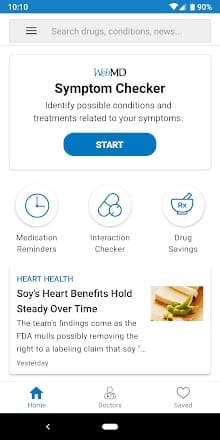At the top of the image, there's a blue rectangle displaying the time "10:10" alongside icons for Wi-Fi, a triangle-shaped symbol, a battery indicator showing "90%," and a notification bell. Directly below this is a gray rectangle housing three horizontal lines on its left side, indicative of a menu icon, and text labels "Search," "Drugs," "Conditions," and "News."

Beneath the gray rectangle, a white rectangle outlined in gray features a prominent "W" followed by the text "WebMD." Below this, in bold black text, it reads "Symptom Checker: Identify possible conditions and treatments related to your symptoms."

Next, there is a unique rectangular button with bulging left and right sides, containing the text "Start." Below this button, there are three white circles outlined in gray with distinct icons inside. The first circle contains a blue clock, labeled "Medication Reminders." The second bears a capsule and pill icon, labeled "Interaction Checker." The third circle has an icon of an Rx with a mortar and pestle, labeled "Drug Savings."

Further down, a white rectangle outlined in gray features the blue text "Heart Health." Underneath this, it reads "Heart benefits hold steady over time," accompanied by an image predominantly featuring brown and green hues, though the exact details are indistinguishable. Below the image, there's a segment of text that is not clearly legible.

At the bottom of the image, a row of icons is present. A blue house icon is labeled "Home," a gray icon resembling a flag inside a circle is labeled "Doctors," and a heart icon with the label "Saved." Lastly, there's a black rectangle with a left-pointing arrow and a white dash, possibly indicating a back button.